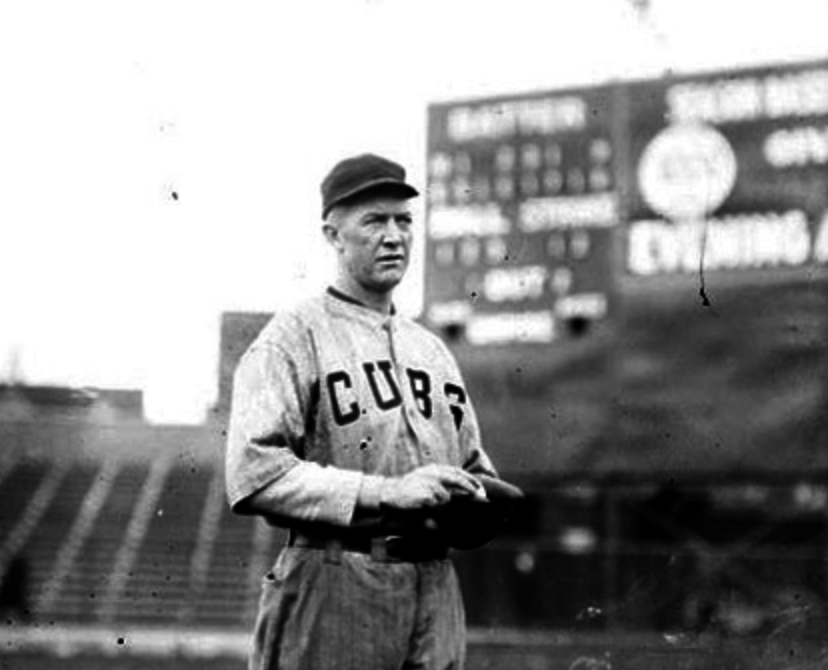This black and white landscape photograph, likely from a bygone era given its poor quality and slight out-of-focus blur, showcases a baseball scene marred by damage to the emulsion with random flakes, tears, and lines. The central focus is a Cubs player in the foreground, wearing period-specific attire including vertically striped trousers, a white undershirt with a pin-striped baseball jersey ending at the elbows, emblazoned with an obscured "Cubs" logo. His dark belt and closely-hugging black cap complete the uniform. The player's left hand appears to hold a catcher's mitt, while his right hand, curled as if gripping a baseball, is engaged with the glove. His neutral expression and gaze are directed slightly to the right. In the blurred background, an empty stadium and a scoreboard with bright, blurred highlights are discernible, along with an indistinct sky. The setting suggests a pre-game or practice moment captured in timeless simplicity.